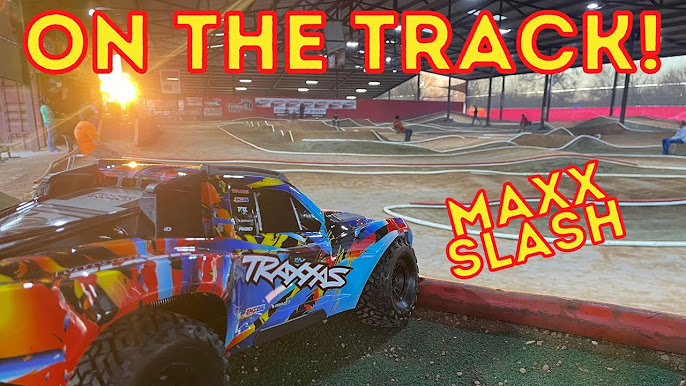The photograph captures a vibrant and colorful race truck, poised on a rugged, multi-leveled dirt track designed for monster truck racing. With large, thickly-treaded tires built for challenging terrains, the truck sports an elaborate exterior adorned with graffiti-like lettering and a bold mix of hues including yellow, orange, red, and black. The track itself does not follow a traditional oval shape, featuring various hills and directional changes for an intense driving experience. Overlaying the image, bold yellow text outlined in red spans the top reading "On the Track," while a slanted caption near the truck reads "Max Slash," presumably the vehicle’s name. In the horizon, seven individuals in brightly colored shirts—red, orange, and green—stand in observance, possibly judges or spectators, with their gazes fixed on the track and its imposing vehicle. The truck is positioned near a red curb on the right side of the image, suggesting it's ready to tackle the course.